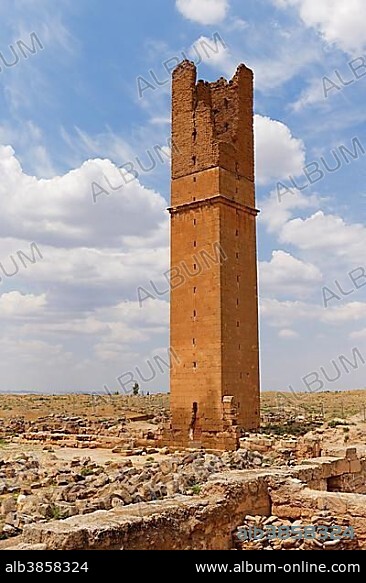The photograph depicts a damaged, tall, rectangular, box-shaped tower in an ancient, deserted, archaeological site. The tower, with a brown-orange hue, stands amidst a bleak landscape filled with fallen bricks and rubble from other demolished stone structures. The top portion of the tower is broken, missing its roof, and exposing its interior with numerous bricks having fallen off. On the right side of the tower, there are two small windows. The clear blue sky above features many white clouds near the ground level. At the bottom of the image, on the left, the text "ALB 3858-324" is visible, while the right side displays "www.album-online.com." Additionally, "ALBUM" is faintly inscribed across the skyline in a diagonal orientation.